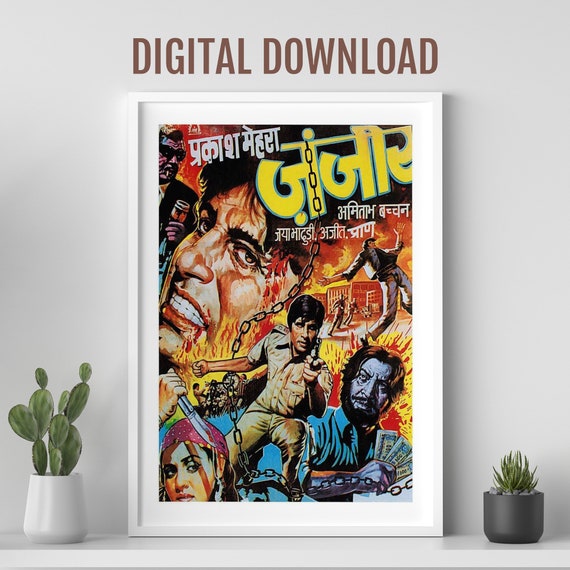The image features a framed poster labeled "DIGITAL DOWNLOAD" in capitalized brown text at the top. The poster, prominently displayed against a white wall and resting on a white shelf, is flanked by two small potted plants: a cactus in a white pot on the left and a succulent in a gray ceramic planter on the right. The poster appears to be an advertisement for an action movie, possibly in a foreign language such as Hindi or Arabic, suggested by the unfamiliar script and yellow and white text.

The poster itself is a dynamic collage of intense scenes. At its center is the main character, a man in a tan uniform with brown hair, aiming a gun directly at the viewer. To his right, a blue-skinned man grips a handful of dollar bills, while flames and chaotic action scenes unfold in the background, including a figure running from a burning building. On the bottom left, a woman with a red or pink bandana holds a knife aloft, her stare fixed on the viewer. The overall composition is punctuated by a chain running vertically through the poster, adding to the sense of tension and drama.